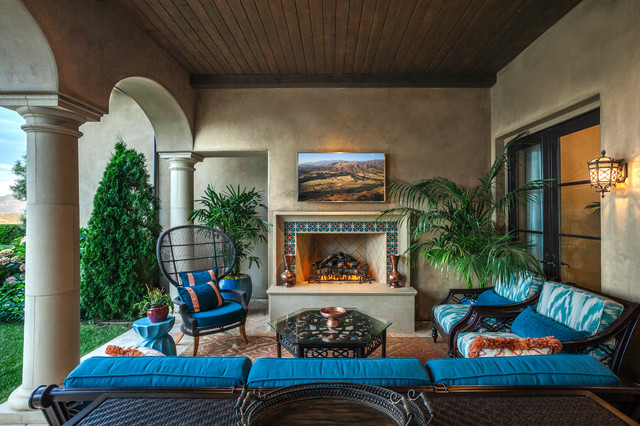This image depicts a charming covered patio area that serves as an outdoor extension of the home, opening to the backyard via an archway supported by elegant columns. The centerpiece of this inviting space is a fireplace adorned with colorful red and blue tiles and framed by cream-colored brick. Above the fireplace, a TV or possibly a pastoral painting enhances the cozy ambiance. Flanking the hearth, two bronze flower pots add a touch of classic elegance.

Directly in front of the fireplace, a wrought iron coffee table with a glass top sits on a large brown rug, surrounded by comfortable rattan furniture. The seating includes a couch and loveseat style chairs with blue cushions, accented by orange highlights and white floral patterns. The deck is covered by a ceiling of rich brown wood, complementing the overall rustic aesthetic. 

To the left, lush vegetation, including a green tree and bushes with vibrant hydrangeas, adds a splash of nature to the scene. The concrete walls and sliding glass doors maintain a sleek, modern look, while the presence of smaller decorative elements like a twisted blue side table, additional plants, and a wall sconce complete the space, creating an ideal setting for both relaxation and entertainment.